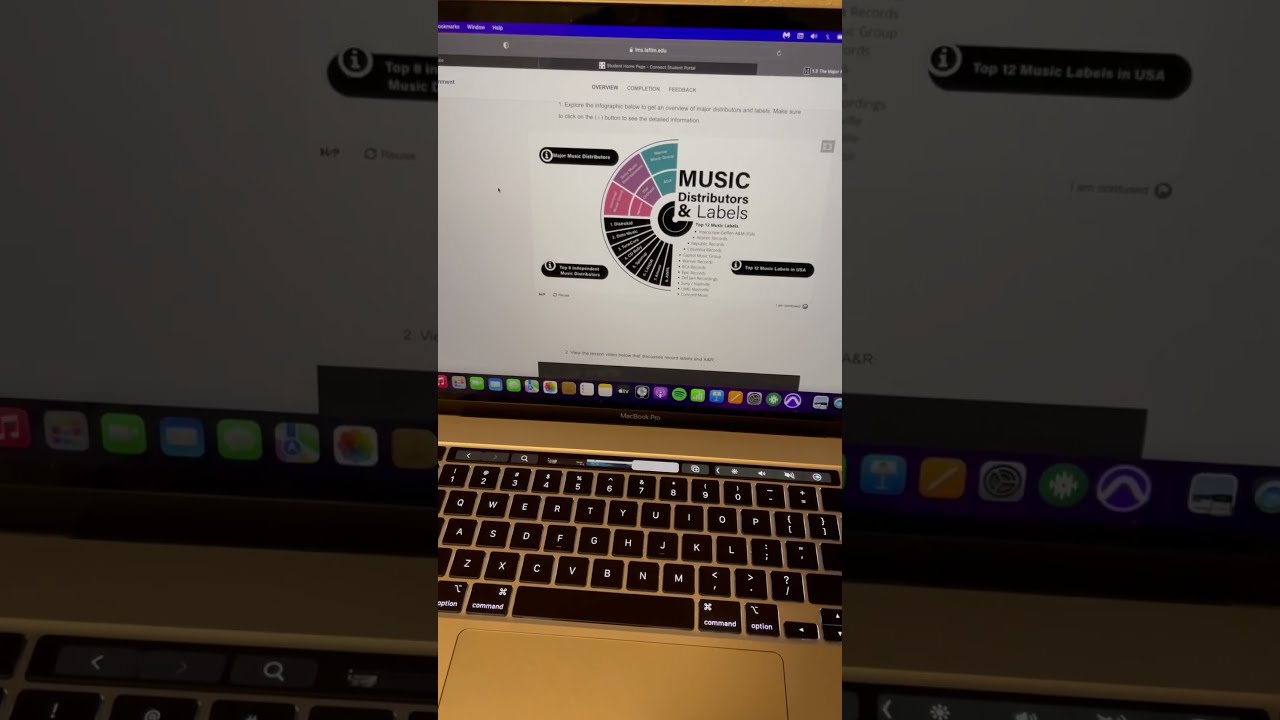The image features a MacBook Pro with a gold metallic finish, displaying a website or application on its screen. The screen prominently shows the text "music distributors and labels," along with an overview section hinting at completion and feedback. The page includes various graphical elements such as half a circle with color-coded sections in green, purple, and pink, accompanied by numbers one through eight, although the specific text in these sections is too small to decipher. The website’s interface primarily uses black text on a white background, highlighted with additional colors like salmon and blue-green. The photograph is taken from the perspective of someone looking at the laptop, with the lower half of the image showing the black keyboard and the upper half displaying the screen’s content. The background of the image appears to be a blurred or enghosted version of the same laptop, adding depth to the picture.